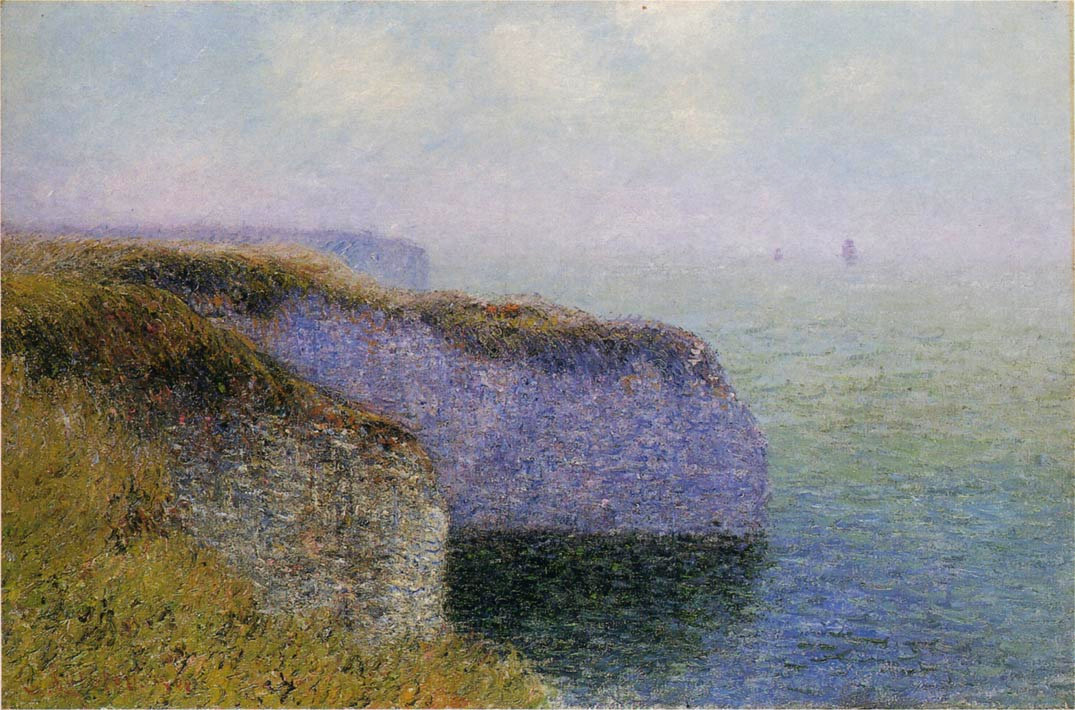This image is an impressionistic seascape, reminiscent of a Monet painting, depicting an expansive body of water—possibly a lake or an ocean—framed on the left by a grassy, foliage-covered hill or series of cliffs. The water itself is a rich blend of greens and blues, with potential hints of boats or distant structures adding subtle intrigue, though these elements remain indistinct. The hill displays hues of green vegetation interspersed with grayish, bluish, and purplish tones, imbuing the landscape with depth and dimension. Above, the sky is a patchwork of blue-gray and lighter blues, scattered with frothy white clouds, suggesting the early to late morning light. The artwork captures a tranquil yet dynamic scene through its meticulous application of dot-like brushstrokes and diverse color palette, featuring various shades of blue, green, yellow, brown, and purple. No people, animals, or textual elements are present, focusing the viewer's attention solely on the serene natural beauty of the scene.